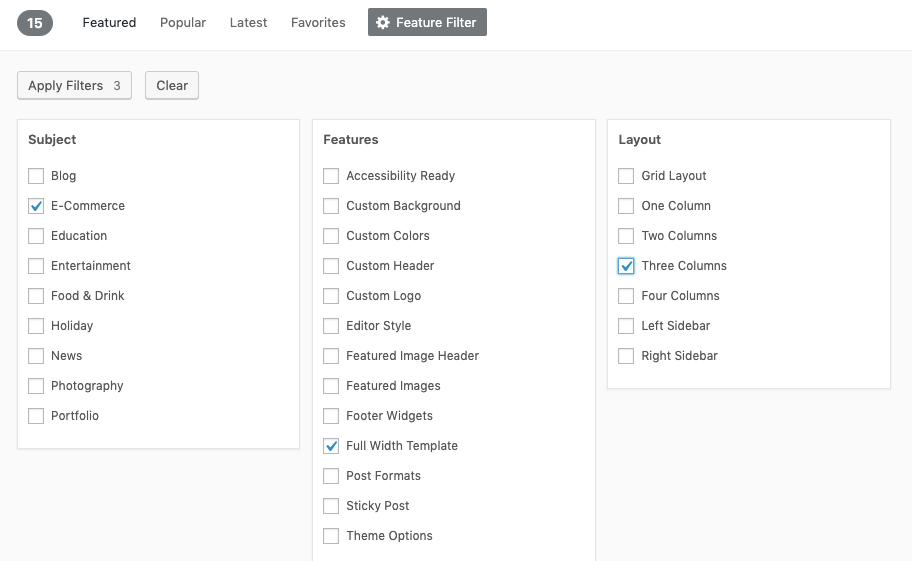In the upper left corner of the image, inside a gray circle, is the number "15." Adjacent to this, the word "Featured" is displayed in gray text, followed by "Popular," "Latest," and "Favorites." To the right, inside a gray rectangle, are the icons for "Feature" and "Filter," with a circle icon next to them. Below this, the text reads "Apply Filters" with the number "3" beside it. Next to this is a box containing the word "Clear."

The first row begins with the word "Subject," followed by approximately eight squares arranged vertically, each labeled with different words. One of the squares has a check mark, and the word next to it is "E-commerce."

To the right, the section titled "Features" consists of about 12 to 13 squares, each labeled with different options. Only one of these squares is checked, next to the label "Full-width Template."

On the far right, under the section titled "Layout," are roughly six to seven choices. The square checked in this section is next to the option "Three Columns." The unchecked options below include "Four Columns," "Left Sidebar," and "Right Sidebar."

The overall layout presents a filtering interface with various options for customizing content categories, features, and layouts, with certain selections indicated by check marks.